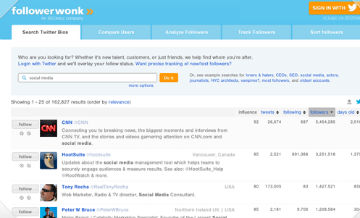This image is a slightly blurry screenshot of a website page, identified as Followerwonk. At the top, there is a prominent blue bar. On the left side of this bar, "Followerwonk" is displayed in white text next to some orange quotation marks. Over on the right, there's an orange rectangular button with white text that reads "Sign in with," accompanied by the white Twitter logo.

Below the blue bar, there are five tabs arranged horizontally. The first tab on the far left is selected, though the exact text is indistinguishable. The remaining four tabs are blue with white text but are too small to read clearly.

Further down, there is a light blue rectangular box containing black text, a search bar, and an orange button adjacent to the search bar. Accompanying this are links in blue, presumably clickable hyperlinks.

The search results below this box show various listings. The top result features a black box with the text "CNN" in red. The second result has a blue background displaying a grey owl wearing sunglasses. The third result is an image of a man with dark hair, also wearing sunglasses, facing left.